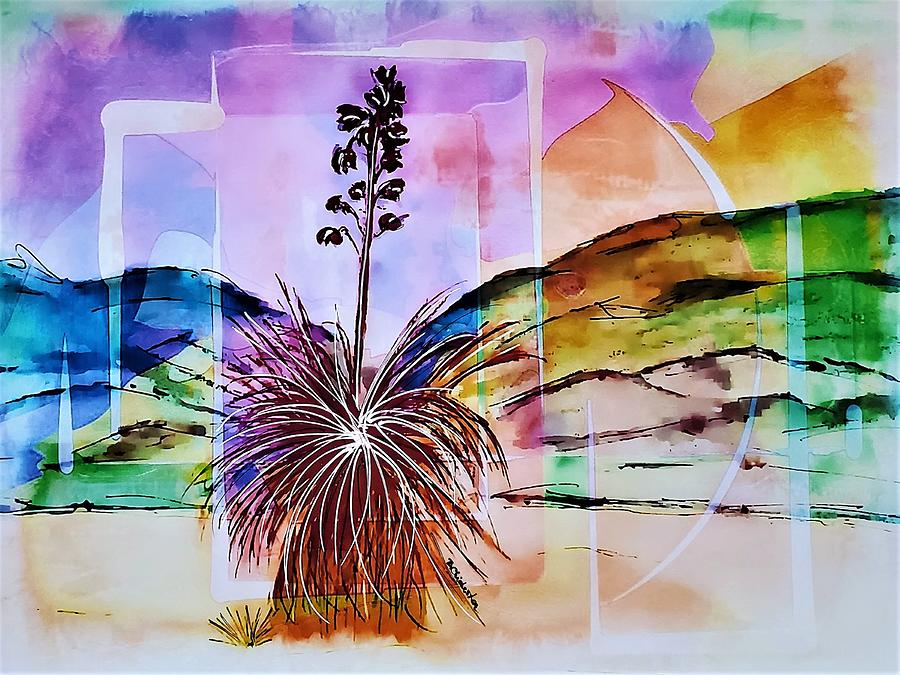This contemporary art piece is a vibrant and colorful print of a watercolor painting depicting a desert scene with various lively hues. The foreground features a striking black and white grassy plant, possibly an agave or century plant, with elongated leaves and a tall stalk adorned with small black buds or berries. The plant appears to be emerging from a wall painted in browns, tans, and peach colors. Surrounding the centerpiece are smaller bunches of grass on a different part of the picture.

The composition includes white rectangles, partial circles, and other geometric shapes scattered throughout, creating a layered effect. Behind the plant, the landscape showcases a series of multicolored hills in blues, greens, dark greens, turquoises, and grays. The sky above is a mesmerizing blend of pinks, purples, peaches, and bronzy tones, adding to the surreal and dreamy quality of the scene. Despite the vibrant chaos, the painting's signature remains illegible, adding a touch of mystery to this captivating piece of modern art.